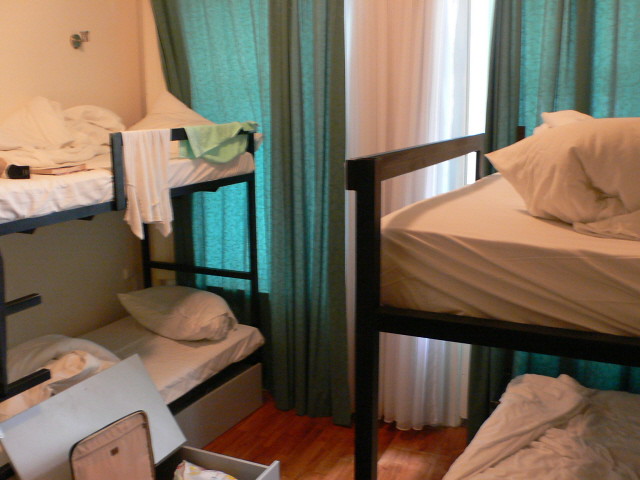The photograph depicts a bright and sunny bedroom with light streaming in from the window on the right, which is adorned with white and green curtains. The room's layout is horizontal, accentuated by a reddish cherry hardwood floor with thin planks. The left wall is white and features two black-framed bunk beds. The bed to the left has a bottom bed with its bedding pulled halfway off, and the top bunk has a crumpled blanket, along with a white towel and green shirt hanging off the edge. Above this bunk bed is an empty wall lamp sconce. On the right side of the room, another set of bunk beds stretches out perpendicular to the first, with both top and bottom bunks displaying disheveled white sheets and pillows. The floor in the bottom left corner showcases a blue chest and a brown item, possibly a bag lid. Additionally, there's an open slide-out drawer beneath the bottom left bunk, suggesting extra storage space. The room's overall arrangement and details reflect a lived-in yet orderly atmosphere.